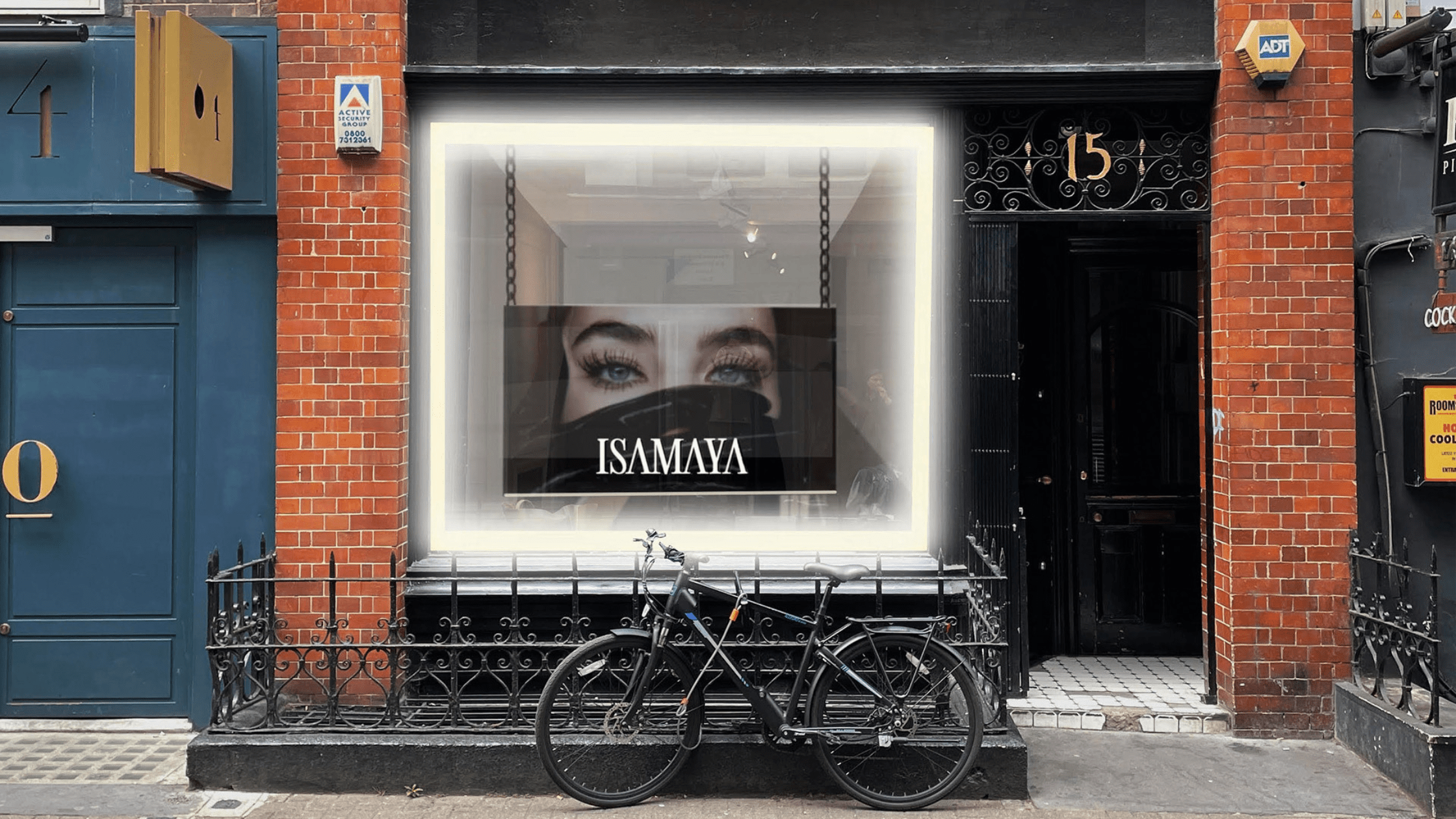The image depicts the front of a couple of storefronts set outdoors on a sidewalk. The main focus is a reddish-brown brick building marked with the number 15, displaying a model named Isamaya in its large window. The model has blue eyes with the lower half of her face obscured, possibly by a black-gloved hand. This storefront also features a prominent black door and is protected by ADT security. In front of the building, there’s a black metal fence with an adult bicycle leaning against it. Adjacent to this building is a bluish storefront bearing the number four, with a gold letter 'O' underlined. A chain-covered or grate-style door appears to the right of the poster, revealing part of a black stairwell. The composition frames the brick columns on either side, contributing to a balanced, wide horizontal view of this business.